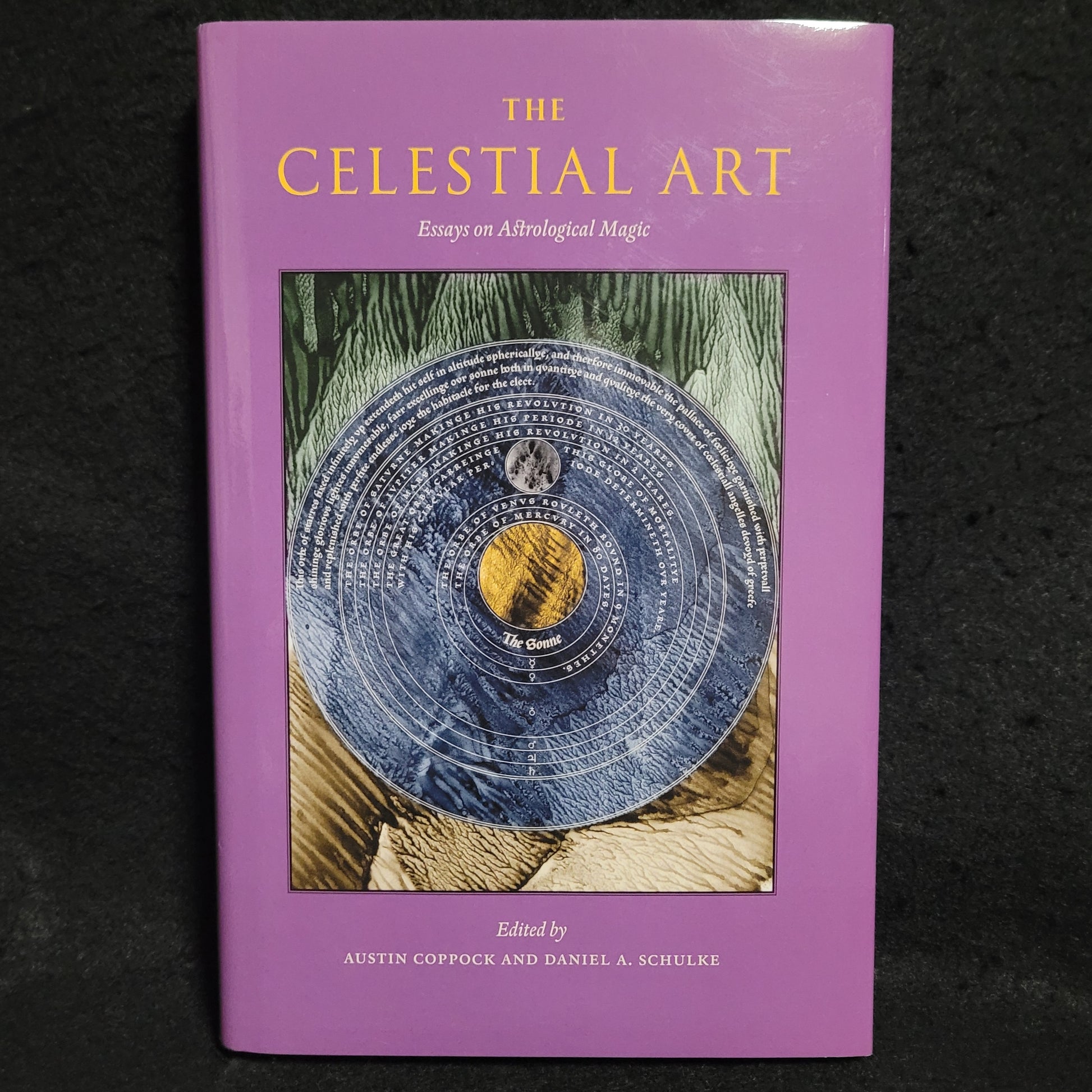This photograph captures a book placed on a solid black surface. The book cover features a light purple background adorned with various elements. At the top, in prominent yellow capital letters, the title reads "THE CELESTIAL ART." Directly below, in smaller white font, the subtitle "Essays on Astrological Magic" is displayed. Positioned centrally is a vertically oriented rectangular image that conceals an astrological chart. Dominating this chart is a large blue circle, reminiscent of a CD, with white text curved around its perimeter and a smaller yellow circle at its center. Behind this circle, an abstract design composed of green mountainous shapes transitions into brown and cream tones toward the bottom. Completing the cover, at the very bottom, in white type, it reads "Edited by Austin Coppock and Daniel A. Schulke."